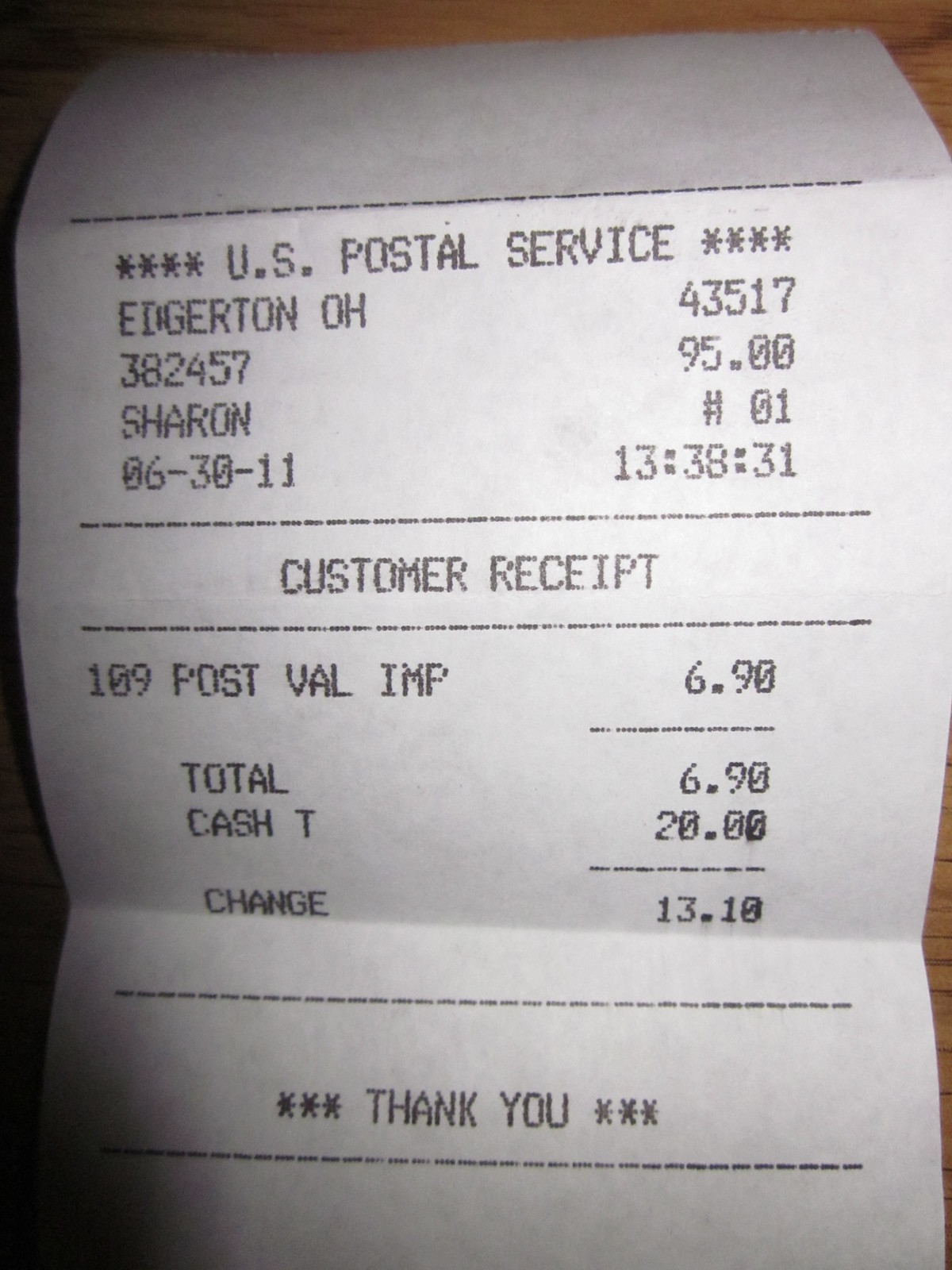This image showcases a slightly folded U.S. Postal Service receipt placed against a wooden background. The receipt's ink is black, and the text proceeds as follows from top to bottom. At the top, surrounded by four asterisks on each side, it reads "U.S. Postal Service." Below this, the location is specified as "Edgerton, Ohio, 43517." Further down, it lists a financial figure: "$382.45/$7.95." The receipt then notes "Sharon #1," which may indicate the cashier or transaction number. A date and time are also present: "06/30/11" at "13:38:31." The section labeled "Customer Receipt" lists a specific transaction - "109 Post Val IMP" costing "$6.90," with a total of "$6.90." The payment method and change are detailed; the purchaser paid with a $20 bill and received $13.10 in change. Finally, the receipt expresses gratitude with "Thank You," flanked by three asterisks on each side at the bottom.